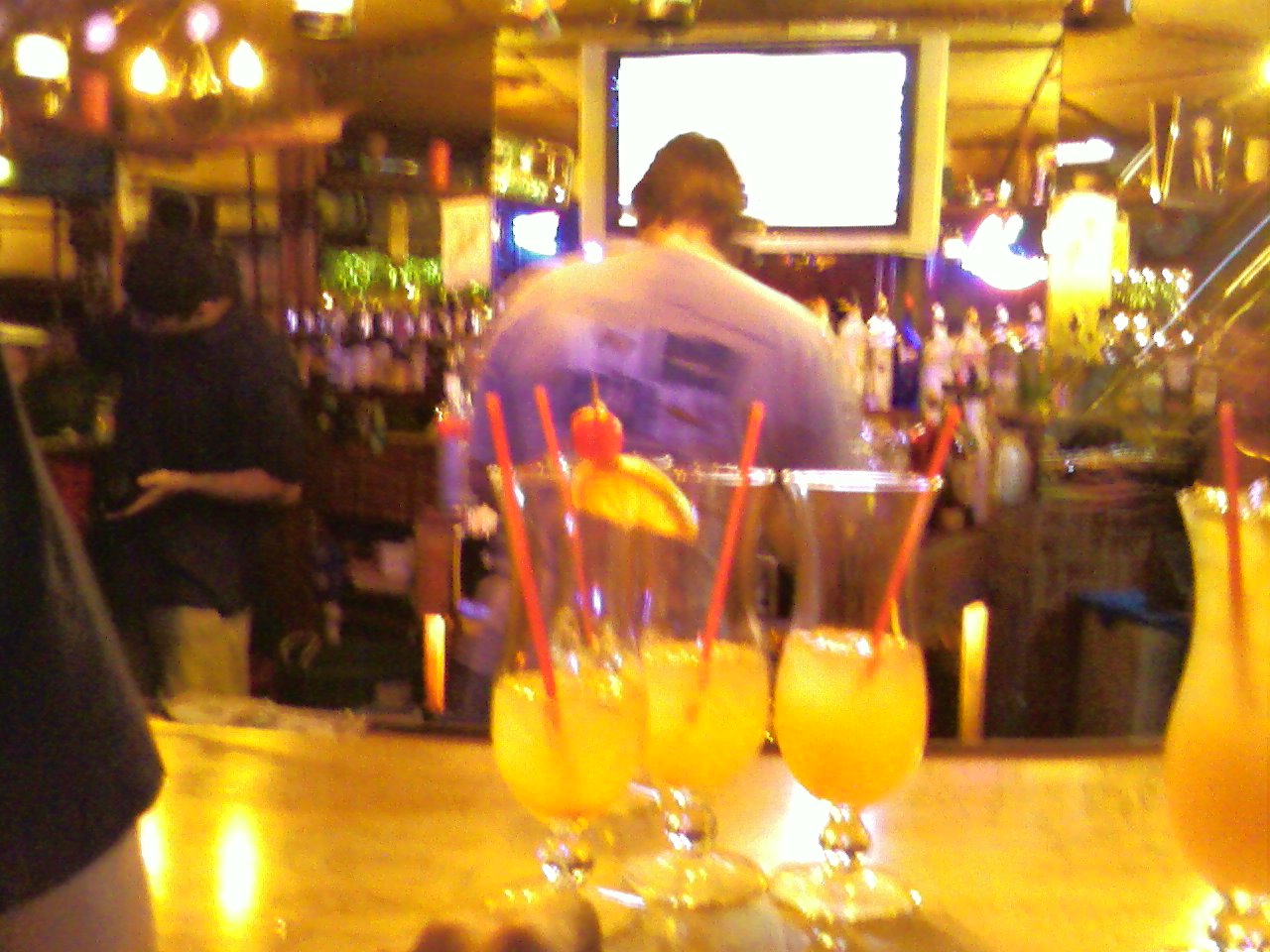In this photo taken at a bar, the image is somewhat blurry and grainy, likely captured with a low-quality cell phone camera. The bar top is a light blonde wood and features four curved hurricane glasses filled with a yellow-orange liquid resembling a tequila sunrise. Each glass is garnished with an orange slice, a cherry, and a pinkish red straw. Behind the bar, there are several details that add to the atmosphere: multiple bottles are stacked horizontally against a mirrored surface lined with lights, and a bright, somewhat overwhelming light from a flat screen TV adds to the picture's overall difficult visibility. The main bartender, who has brown hair and is wearing a light purple shirt with a logo on it, is positioned in the center, appearing to be working at a cash register. Off to the left, another bar staff member in a black t-shirt and gray pants can be seen assisting customers.